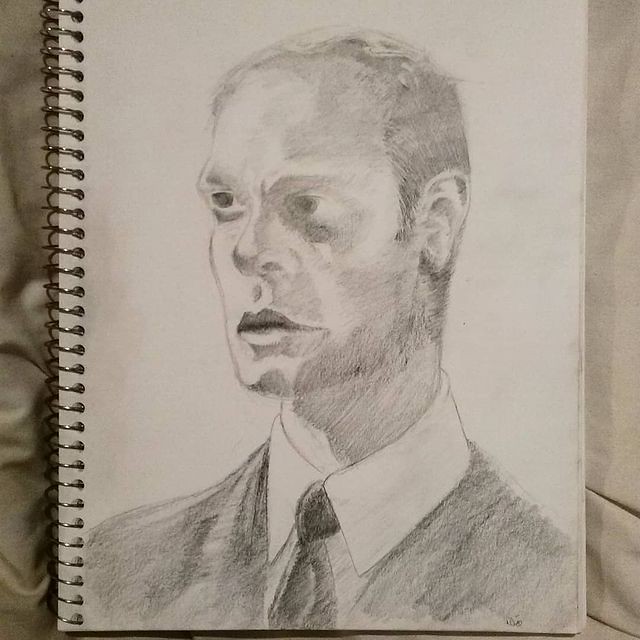This image features a detailed charcoal or pencil sketch mounted on a spiral-bound sketch pad, angled against what appears to be a pillow or couch cushion. The visible spiral binding on the left side of the pad adds a sense of authenticity to the artist’s workspace. The sketch itself is a highly expressive portrait of a man, focusing on his head and shoulders. The subject has very short hair, neatly parted to the side, and is dressed formally in a suit, tie, and crisp white collared shirt. Notable facial features include a sharp jawline, full lips, high cheekbones, and a slender face. His eyes draw particular attention; while one eye gazes intently straight ahead, the other eye appears slightly misaligned, with the pupil turned inward towards the inner corner, suggesting a touch of a lazy eye. The portrait exudes character and meticulous craftsmanship, capturing the subtleties of the man’s expression and demeanor.